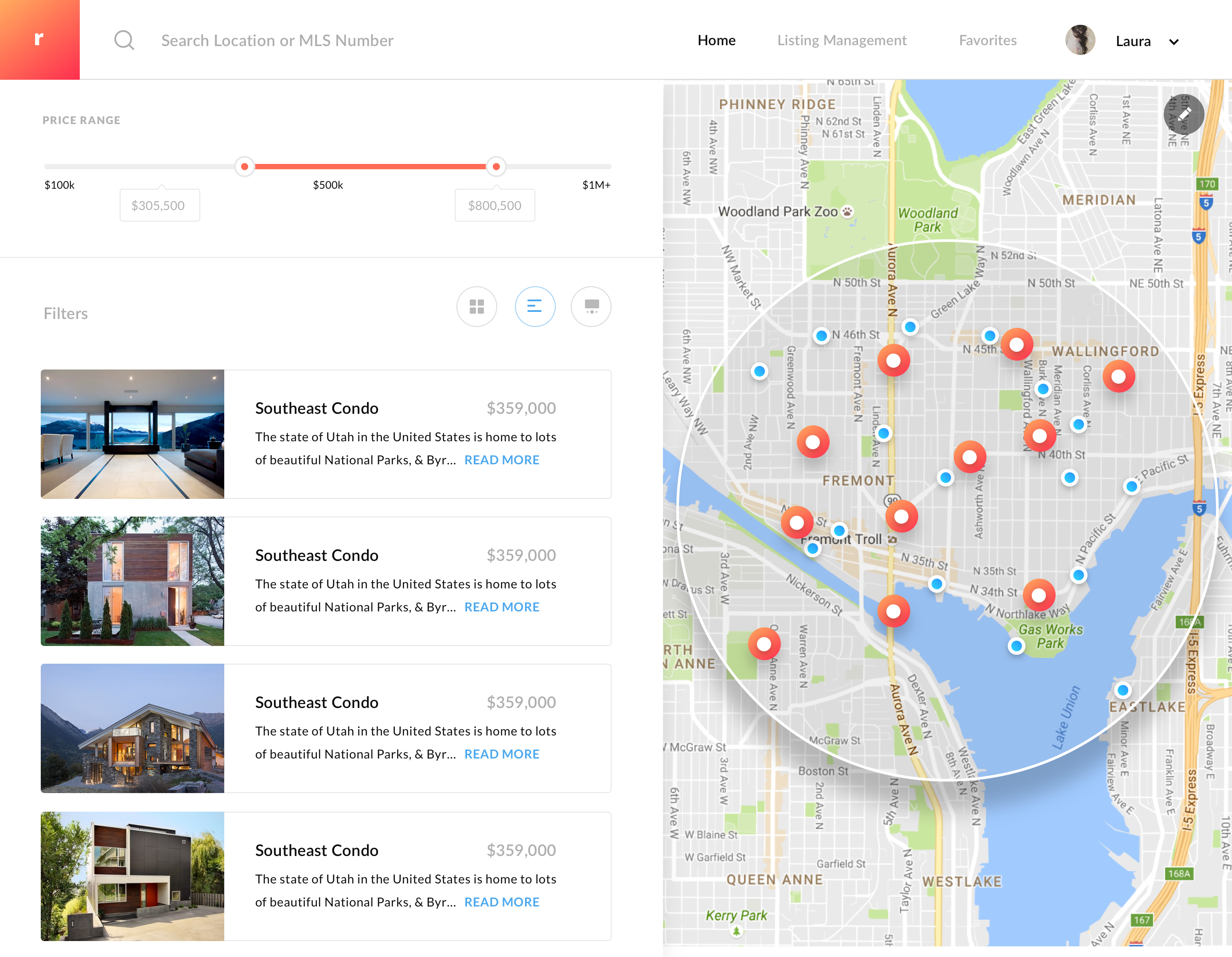The image displays a website interface for a real estate platform. Prominently, there's an "R" inside a red box at the top. Adjacent to it is a search bar followed by navigational links labeled "Home," "List," "Management," "Favorites," and "Laura." The "Home" and "Laura" links are highlighted in dark black, indicating they are selected or currently active. 

Next to the name "Laura" is her profile picture. Beneath this navigation bar, the site shows a price range marker illustrating home prices from $100,000 to $1,000,000. A red indicator bar hovers around the $500,000 mark, and there are boxes showing specific price points at $305,500 and $805,000.

Below the price range indicator, there is a "Filters" button that users can click to refine their search criteria. The site currently lists several condos for sale, all located in the Southeast region. The condos are uniformly priced at $359,000, although there are stylistic differences: three of them are categorized as modern and one as contemporary.

A large map is embedded on the site, displaying pins that mark the locations of all the listed properties. Additional listings are noted beyond the initial ones provided, offering users further options to explore.